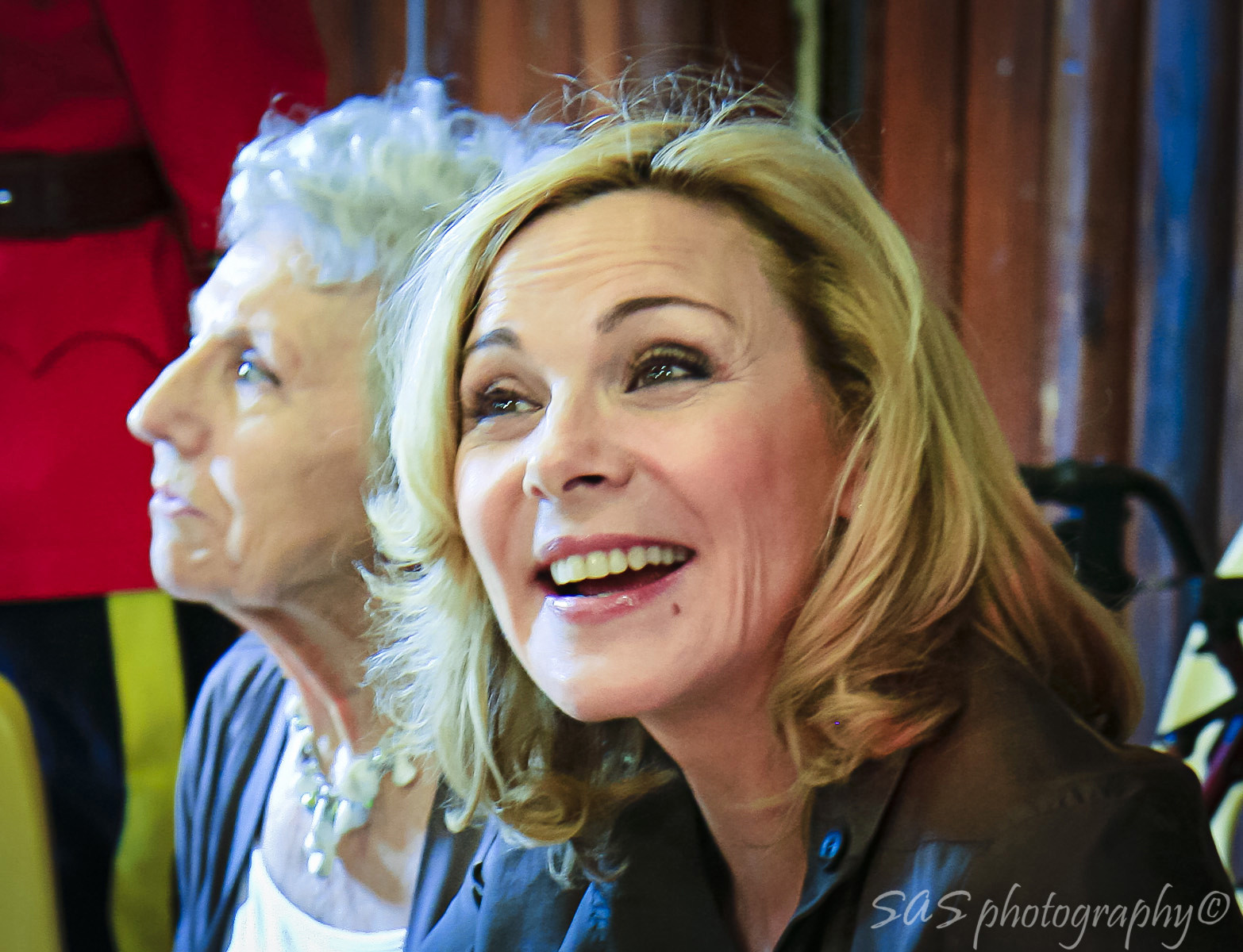The image, taken by SAS Photography, features a close-up of two women, both of light complexion, capturing their faces and shoulders. The woman on the right, who appears middle-aged, has short blonde hair and is wearing a black top. She is seated and smiling, looking up engagingly as if in conversation. To her left is an older woman, possibly her mother, with short white hair. She is adorned with a costume jewelry necklace over a white scoop-neck shirt, layered with a blue jacket. This older woman is also looking to the left of the image. The background reveals an indistinct, colorful backdrop, perhaps curtains or a wall, with a hint of a person in a bright red jacket and black belt partially visible. The overall setting is brightly lit, presumably by natural light, enhancing the vibrant and engaging atmosphere of the scene. The bottom right-hand corner of the image is marked with "SAS Photography" along with a copyright symbol.